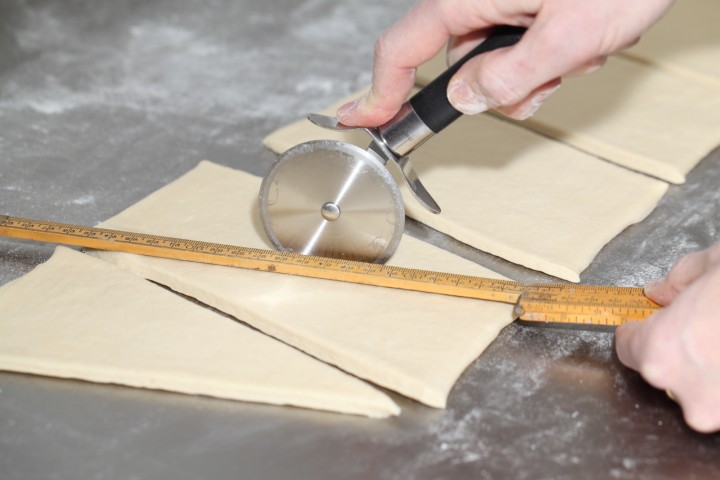In the photograph, which is rectangular with the top and bottom sides twice as long as the left and right sides, a person is meticulously cutting pastry dough on a stainless steel countertop dusted with white flour. Only the person’s hands are visible; their left hand holds a slightly bent wooden ruler to guide their precise movements. Their right hand maneuvers a pizza cutter with a blade coated in white powder. The person is carefully slicing the rectangular-shaped pastry dough into triangular pieces, using the ruler to ensure accuracy. Multiple rectangular dough pieces are lined up in a row, with a neatly cut triangle already visible in the bottom left corner. The dough has a light yellow hue, contrasting with the silver work surface underneath. The methodical process and the setup suggest a focused effort to achieve a specific shape, possibly for a future culinary creation.